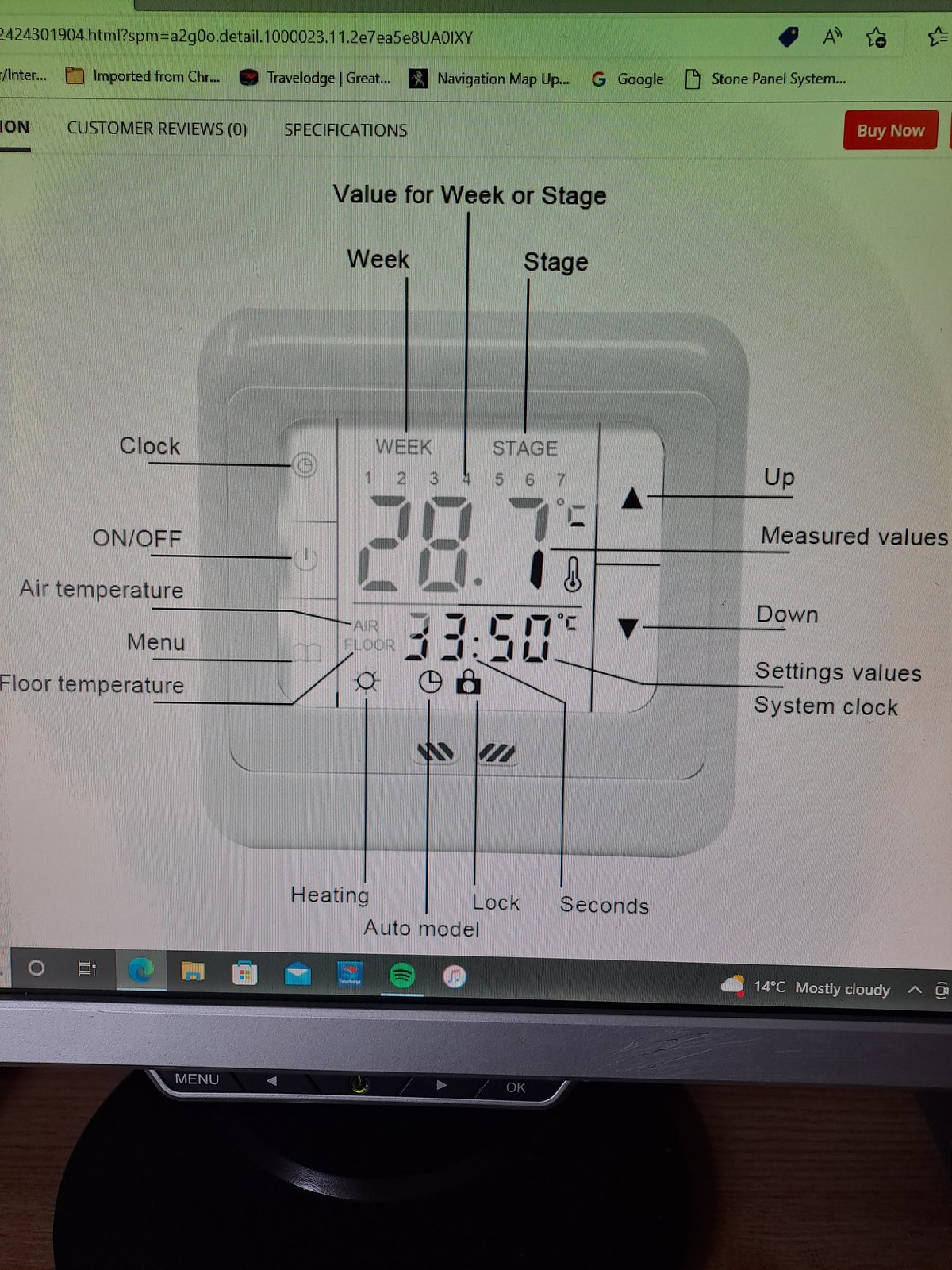This color photograph captures a close-up view of a computer monitor screen displaying a webpage. At the top, the browser’s address bar and a few favorite links saved on the toolbar are visible. The central focus of the screen is a detailed diagram, presumably of a thermostat or clock, enclosed in a gray square casing with an LCD screen. The LCD screen displays a temperature reading of 28.7°C prominently in the center, and a secondary reading of 33:50°C below it.

Various parts of the thermostat/clock are labeled across the screen with terms such as "value for week or stage," "Week," "Stage," "Clock," "On," "Off," "Air temperature," "Menu," "Floor temperature," "Heating," "Auto mode," "Lock," "Seconds," "Up," "Measured values," "Down," "Settings values," and "System clock." 

In the top right corner of the screen, a red square button labeled "Buy Now" in white text draws attention. To the top left corner, the options "Customer Reviews" (with a zero in parentheses) and "Specifications" can be seen.